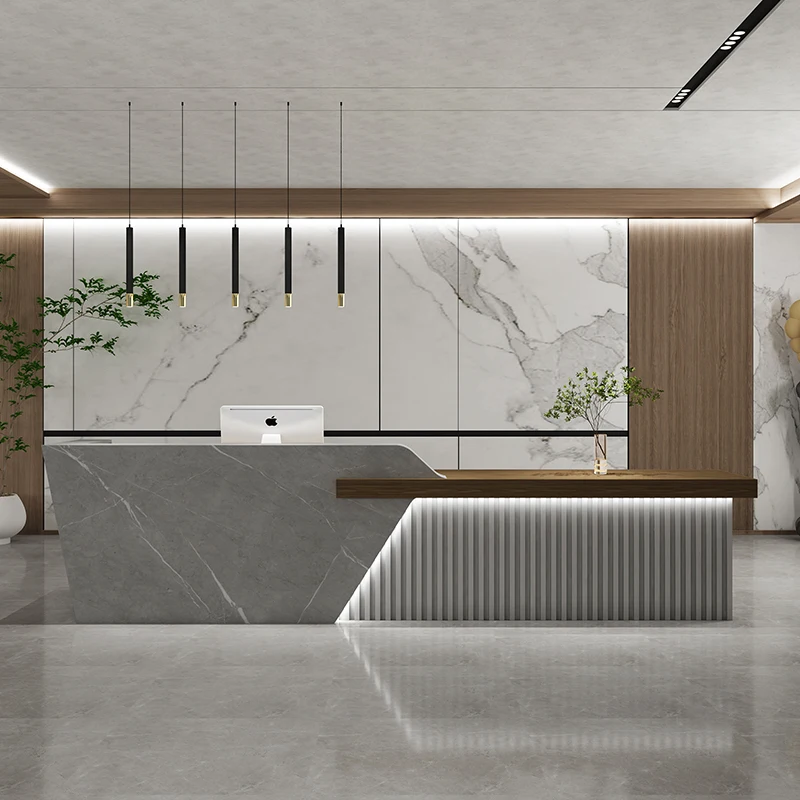This is a detailed 3D color illustration of a modern business reception area, created in an application like SketchUp. The room features a highly reflective dark gray marble floor that mirrors various pieces of furniture throughout the space. The back wall showcases an elegant combination of large white marble panels interspersed with dark brown wood accents, creating a striking visual contrast. The ceiling is painted white, equipped with recessed bar lighting, along with black string lights that have alternating black and white fixtures hanging from them.

At the center of the room is a contemporary reception countertop, which has a sophisticated design: the left side is crafted from gray marble, while the right side features ridged white paneling topped with a thick brown wood block. This wooden countertop section supports a white Mac computer monitor, with the recognizable Apple logo facing the viewer. On the same countertop, there's a round clear vase holding a green branch.

In the foreground, the reflective gray marble floor continues to enhance the room's modern aesthetic. The overall effect is a meticulously designed, highly detailed space that blends modern materials and thoughtful lighting to create an inviting yet professional atmosphere.